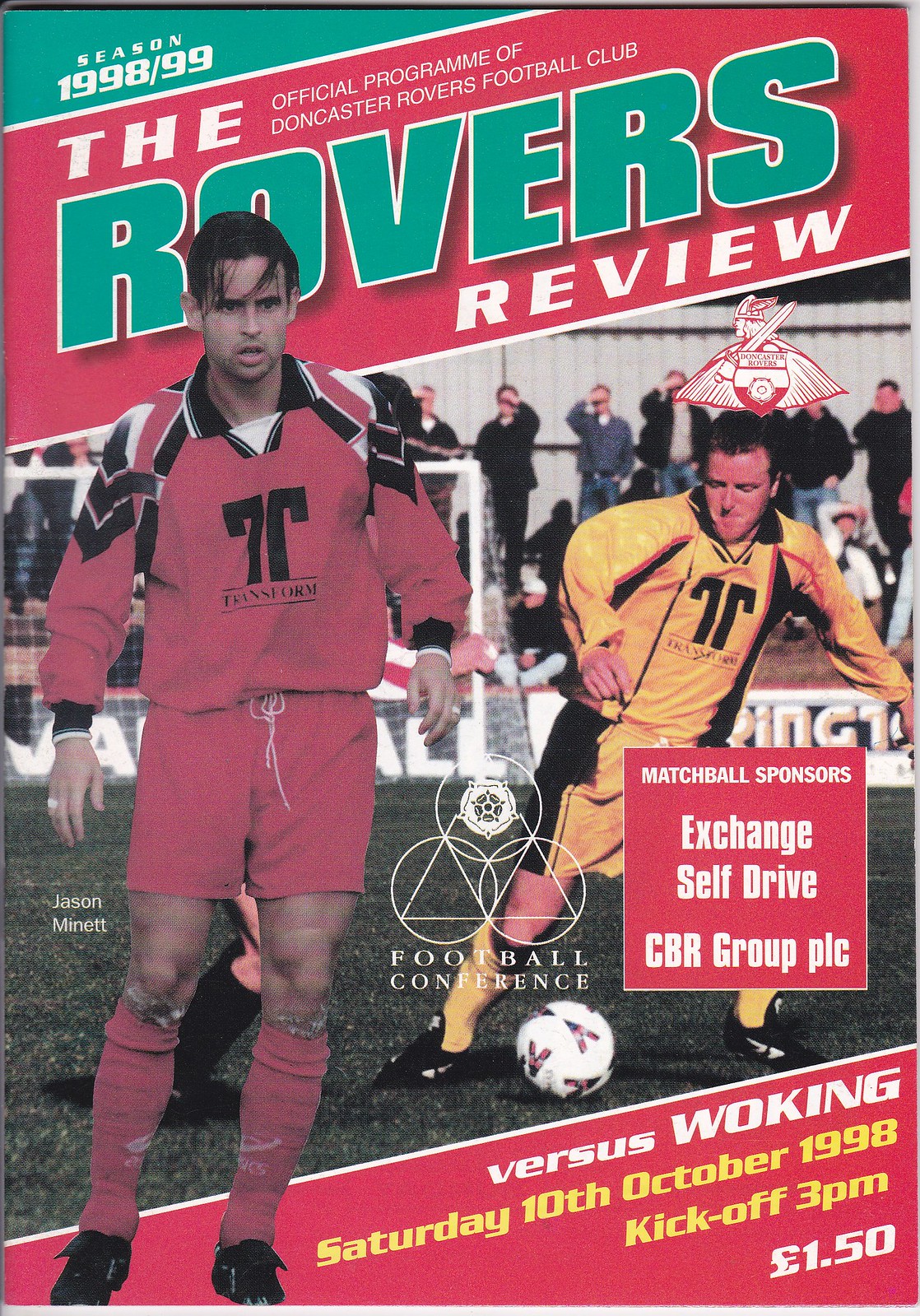This is the cover of the Rovers Review magazine for the 1998-99 season, the official program of the Doncaster Rovers Football Club. The title "Rovers Review" is displayed prominently in green bold font, with "The" and "Review" in slightly smaller white font across a red band in the upper left corner. Smaller text underneath reads "Official Program of Doncaster Rovers Football Club". 

At the center of the cover are two soccer players overlaid against each other. The player on the left is dressed in a long-sleeve red top, red shorts, red socks, and black shoes, with black hair, while the player on the right is in a long-sleeve yellow top, yellow shorts, yellow socks, and black shoes, standing next to a white soccer ball. Both are wearing jackets, and the background shows spectators watching the match.

In the middle of the image, there is a triangle with three circles and the text "Match Ball Sponsors Exchange Self-Drive CBR Group PLC Football Conference". 

In the lower right-hand corner, there is a red band stating, "vs. Woking, Saturday, 10th October 1998, kickoff 3 p.m., £1.50".